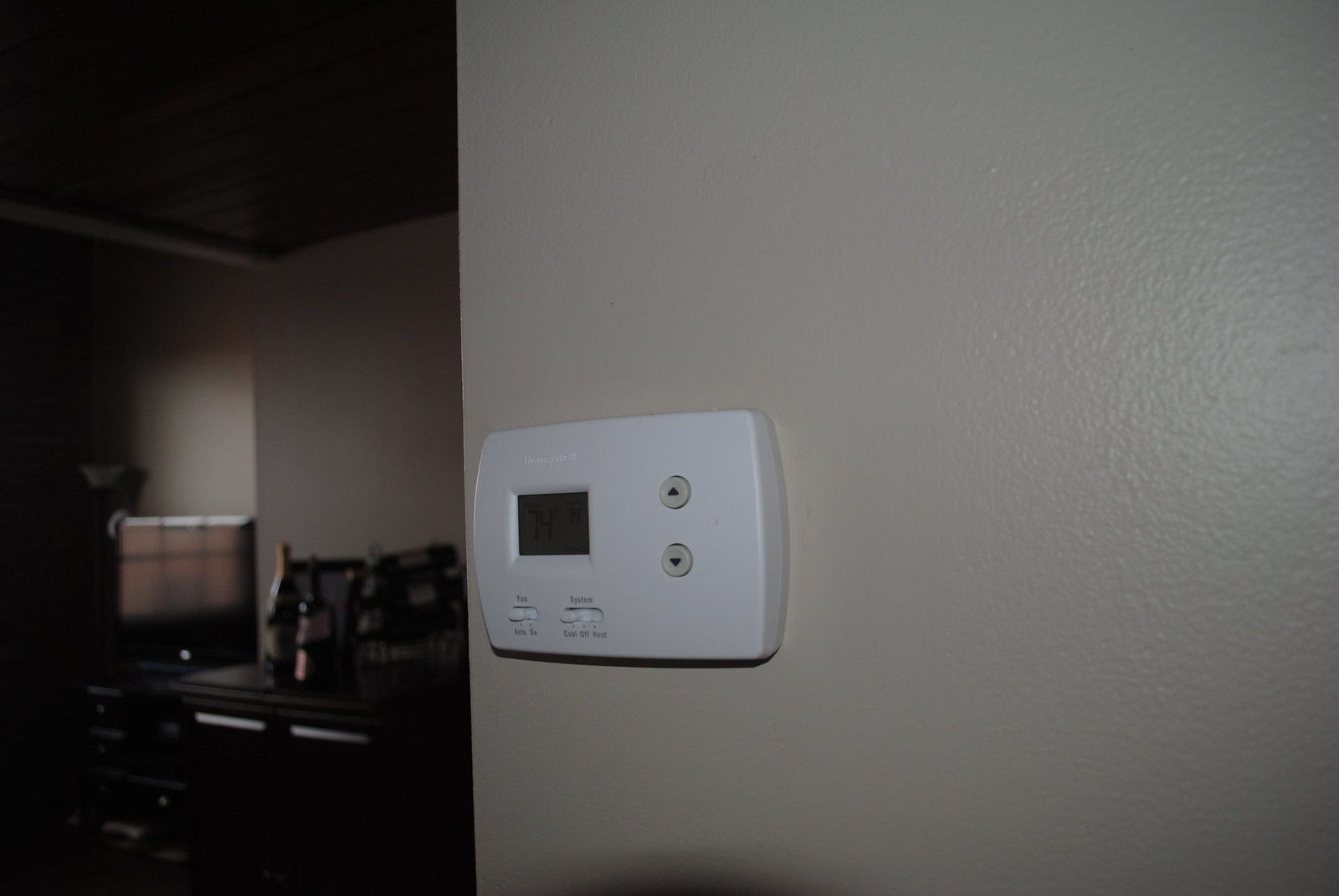A dimly lit room reveals a wooden desk adorned with two bottles of wine, positioned strategically in the center. The scene is set against the backdrop of an adjacent hallway, adding depth to the image. On the right side of the frame, a close-up view of an off-white wall showcases a thermostat for controlling the air conditioning. The white plastic device features clear up and down buttons for regulating the temperature, providing a subtle yet functional touch to the overall ambiance of the room.